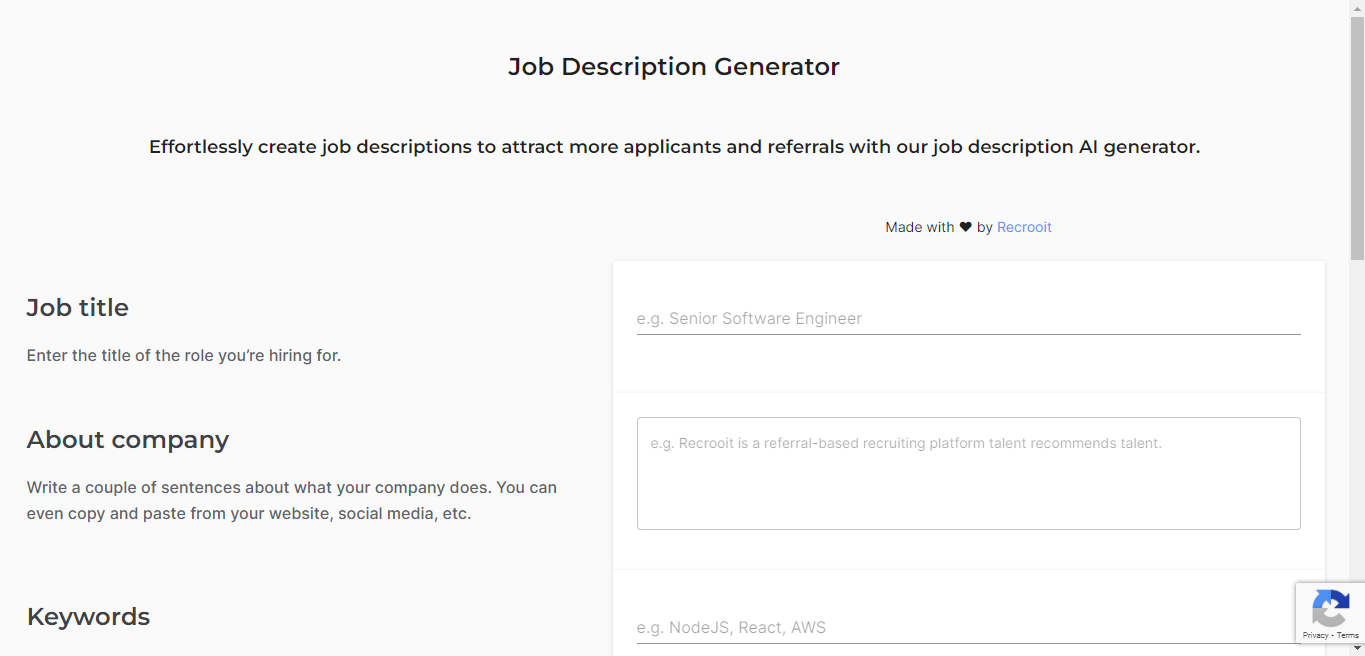This image showcases a webpage designed for generating job descriptions. At the top, the header prominently reads "Job Description Generator." Below this, a subheading states, "Effortlessly create job descriptions to attract more applicants and referrals with our Job Description AI Generator." The text also includes a note, "made with ❤️ by recruit," indicating the developers' identity and effort.

Underneath, there is an interactive field labeled, "Enter the title of the role you're hiring for," where users can input the job title they seek to fill. Further down, a section titled "About Company" invites users to write a brief description of their company, encouraging them to copy and paste relevant information from their website, social media, or other sources. An example within this section reads, "e.g. recruit is a referral-based recruiting platform. Talent recommends talent."

Another field, labeled "Keywords," prompts users to enter keywords relevant to the job role, such as technological skills or software proficiencies. An example provided in this section lists, "Node.js, React, and AWS." 

At the bottom corner of the page, a reCAPTCHA symbol is present, featuring a couple of blue arrows and one grey arrow, accompanied by the words "Privacy" and "Terms," ensuring users' submissions are secure and compliant with privacy standards. The overall design is set against a grey background and includes various fields where users can enter the necessary information to generate a comprehensive job description.